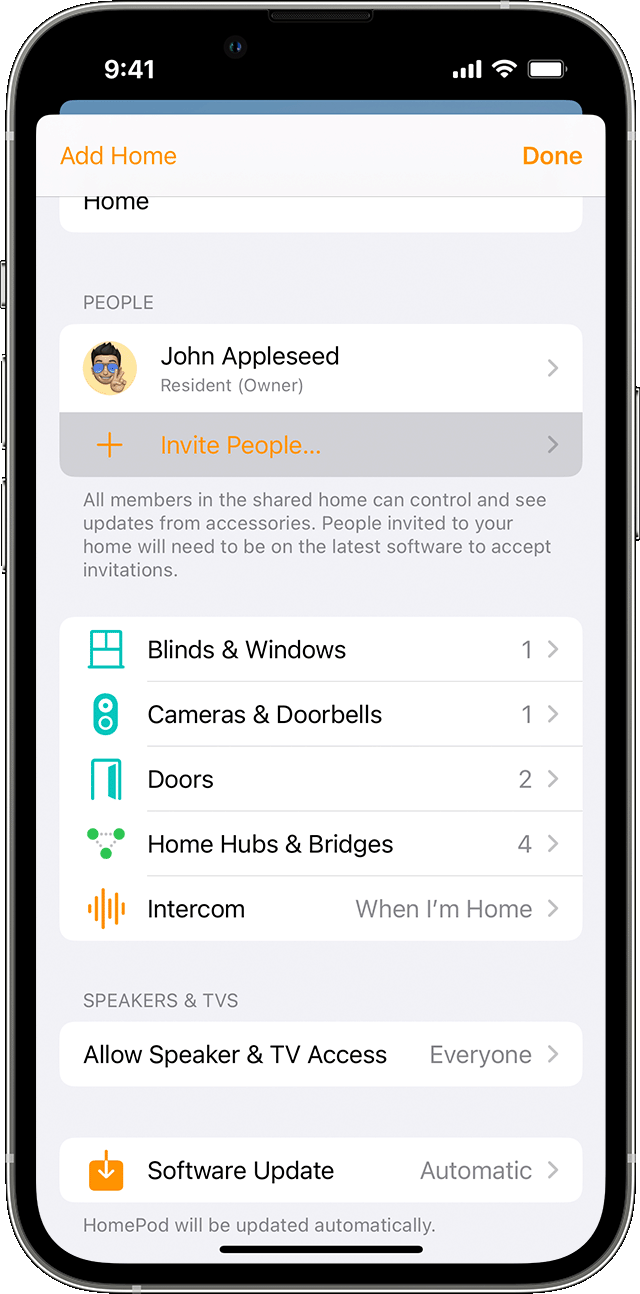This image showcases the front of an iPhone enclosed in a sleek, silver case with three buttons visible on the left side and one on the right. The iPhone screen displays the Settings app, specifically a screen related to home settings. At the top right corner of the screen, there are orange-colored options labeled "Add Home" and "Done". The background of the settings menu is gray.

Under the header "People," there is a highlighted box that reads "John Appleseed, Resident Owner." Below that is a dark gray box indicating the option to "Invite People." 

Underneath these boxes, a message explains: "Members in the shared home can control and see updates from accessories. People invited to your home will need to be on the latest software to accept invitations."

Further down, there are several components listed with accompanying icons and numbers that denote the count of each item:
1. "Blinds and Windows" – represented by a window icon and the numeral "1."
2. "Cameras and Doorbells" – indicated with an appropriate icon and the numeral "1" with an arrow pointing to the right.
3. "Doors" – symbolized by a door icon and the numeral "2."
4. "Home Hubs and Bridges" – illustrated with an icon and the numeral "4."

Following these lists, there are additional categories:
- "Intercom," featuring an icon and an option labeled "When I'm Home" to the right.
- "Speakers and TVs" with further settings listed beneath it.
- At the very bottom, there is an option for "Software Update."

Every detail on the screen has been meticulously organized to ensure ease of navigation and clarity for the user.